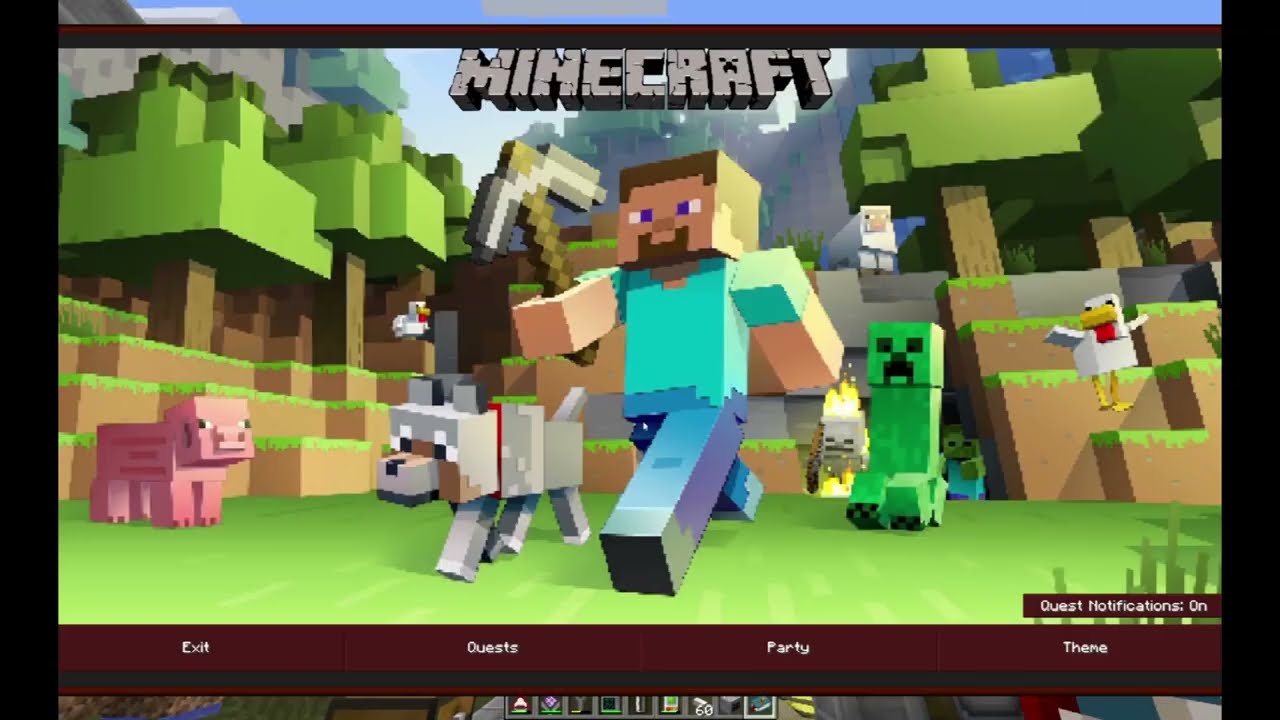The image depicts a vibrant and detailed Minecraft scene set as the main menu screen of the game. Across the top center, large, three-dimensional grey text reads "MINECRAFT." The bottom of the screen features a dark brownish-red menu bar with white buttons labeled EXIT, QUESTS, PARTY, and THEME, accompanied by a small box stating "QUEST NOTIFICATIONS ON."

The scene within the menu illustrates a diverse and bustling Minecraft landscape. The central figure is the main character, a bearded man with brown hair, wearing a teal shirt and blue pants. He is running to the left, holding a pickaxe and accompanied by his grey dog with brown around its muzzle and a red collar. In the foreground, there are two chickens—one on either side of the character. To the left, a pink pig can be seen, while a white sheep stands on a small hill behind him. Menacingly close are several green creepers, a zombie, and a skeleton wielding a flaming bow.

The backdrop showcases an array of blocky, pixelated features typical of Minecraft. There are mountainous areas and cliffs topped with green grass and brown soil underneath. The landscape comprises various trees with blocky trunks and foliage. The entire scene captures the essence of Minecraft's distinctive visual style, emphasizing its pixelated, block-based art.